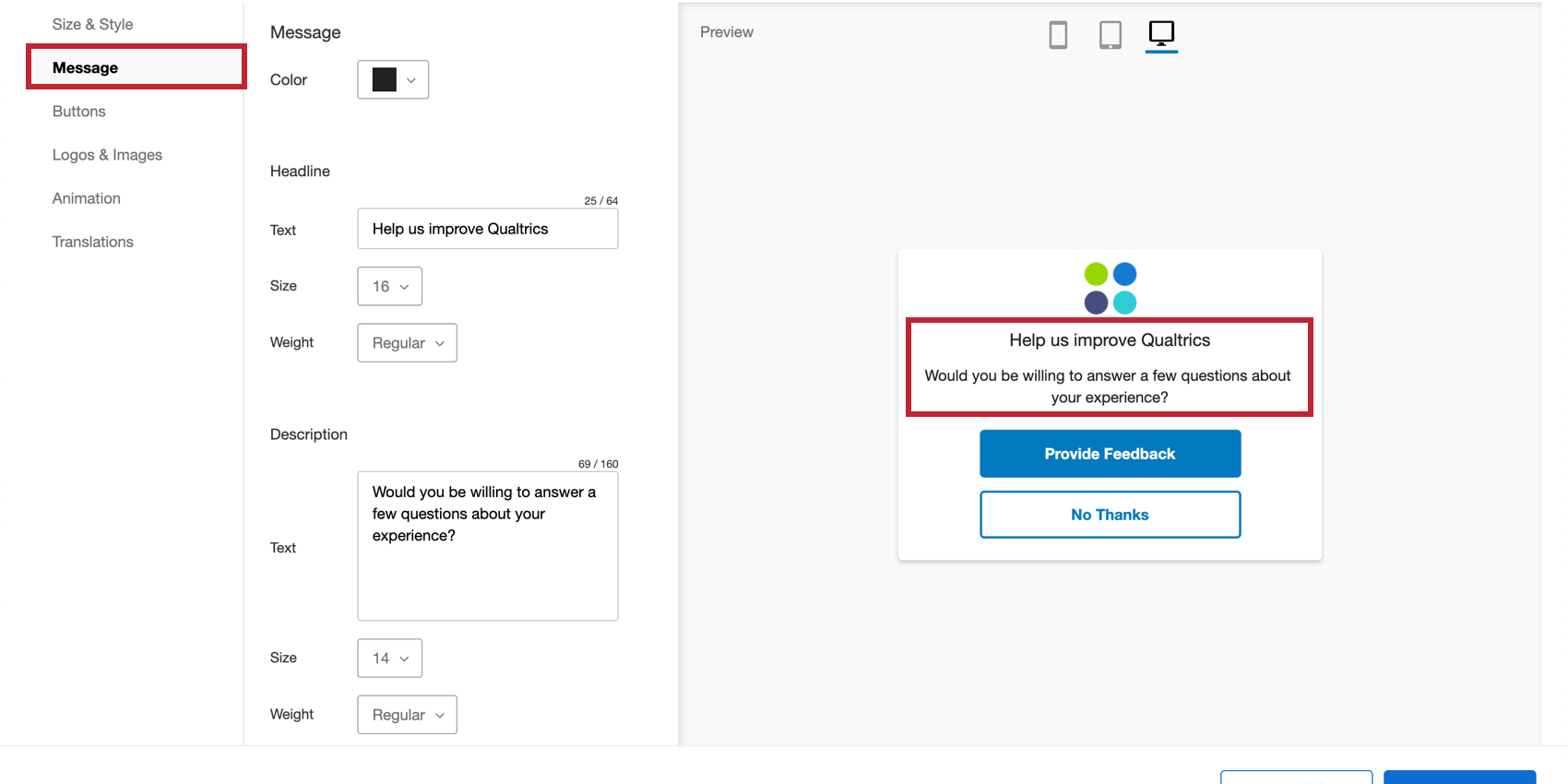This image depicts a user interface page from Qualtrics dedicated to customizing size and style settings. At the top, there are multiple tabs labeled "Messages," "Buttons," "Logo and Images," "Animation," and "Translations," providing different customization options. 

To the right, there is a section to edit a message where users can choose the color of the text and headline, with current text stating, "Help us improve Qualtrics." Below this, options for adjusting the font size and weight are provided through drop-down menus. Another message section below includes the text, "Would you be willing to answer a few questions about your experience?" with similar customization options for font size and weight.

On the right side of the page, there's a preview pane allowing users to see their changes in real-time. Icons to switch between views for a computer screen, tablet, and smartphone are visible, with the current preview shown in the computer screen view.

A pop-up box in the center of the preview contains four dots in green, blue, black, and sky blue colors. A red circle highlights the query, "Help us improve Qualtrics. Would you be willing to answer a few questions about your experience?" Below this message, there are two buttons: "Provide Feedback" and "No Thanks."